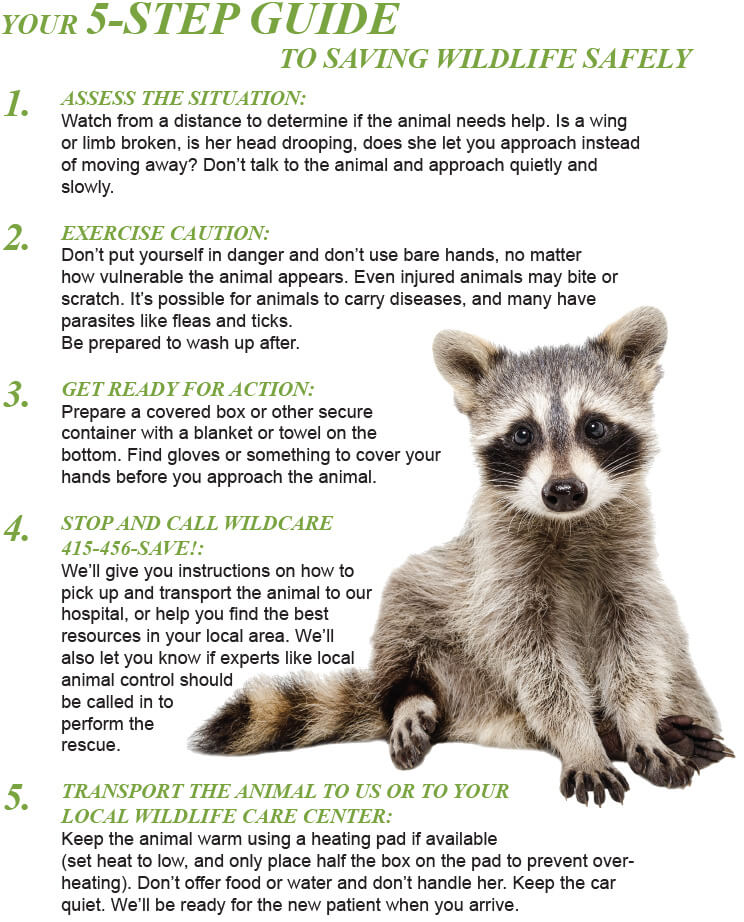The image showcases a detailed, five-step guide on how to safely save wildlife, prominently displayed on a white background. The guide's title, "Your Five-Step Guide to Saving Wildlife Safely," is written in green text, with each step also highlighted in green, followed by detailed instructions in black text.

1. **Assess the Situation**: Observe carefully to determine if the animal needs help.
2. **Exercise Caution**: Do not endanger yourself. Injured animals may bite or scratch and can carry diseases. Use gloves or protective clothing before approaching.
3. **Get Ready for Action**: Prepare a suitable container and wear protective gear. Have a means of self-defense if necessary.
4. **Stop and Call WildCare (415-456-SAVE)**: Get instructions and local support if available.
5. **Transport the Animal**: Keep the animal warm using a heat pad, do not give it food or water, and transport it quietly to WildCare or a local wildlife care center.

The guide includes an illustrated example of a baby raccoon with a gray and tan coat, black-pawed tips, a dusting of black on its head, black stripes over its eyes, a black nose, white mouth, and a black-and-tan striped tail.